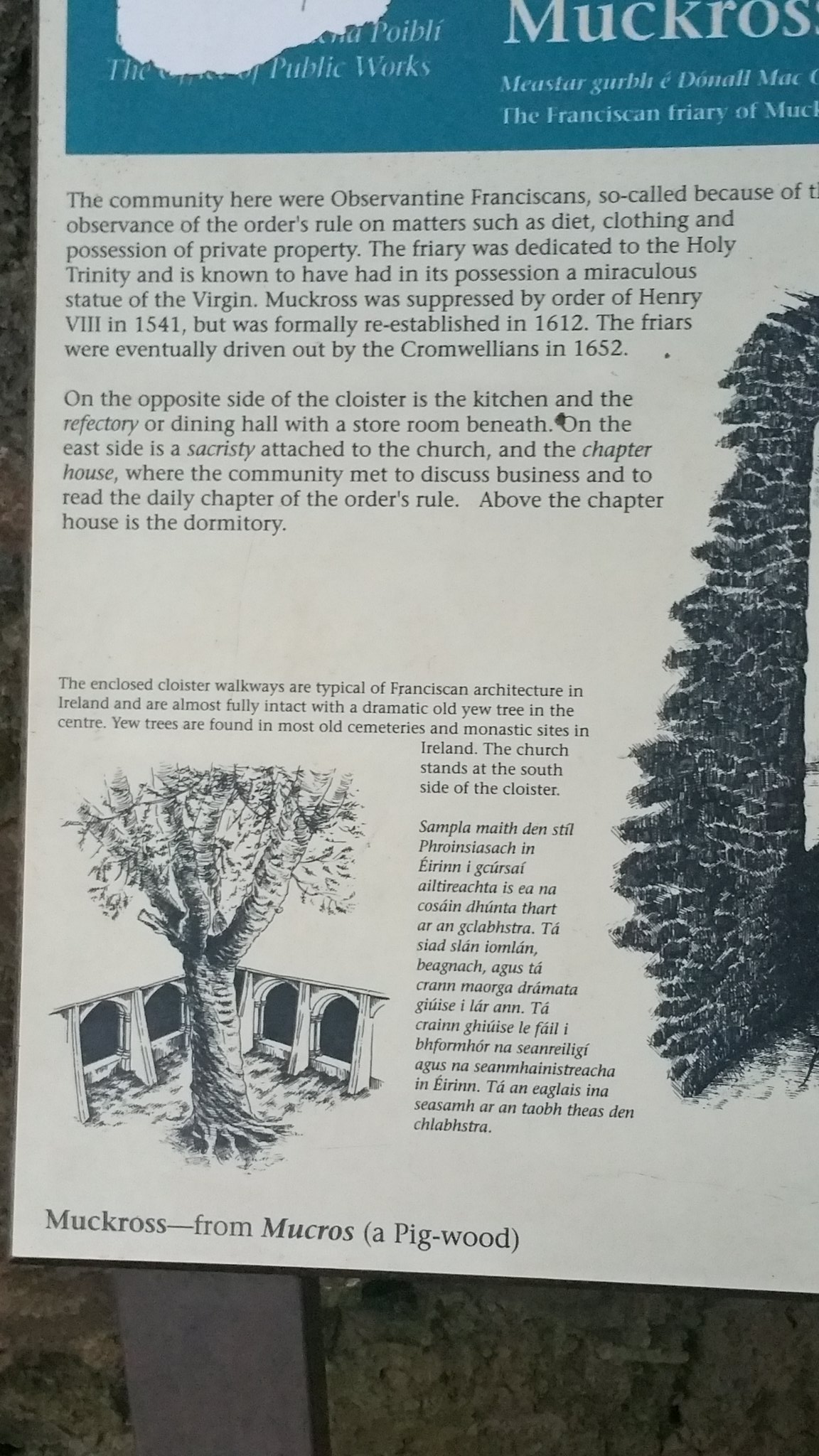This photograph captures a vertically aligned rectangular poster placed outdoors, partially cut off on the right side. The poster, mounted on what appears to be a wooden pole, stands against a background that includes some stones and an unclear structure. The top section features a white background with a blue horizontal strip containing the partially visible word "Muckross" (M-U-C-K-R-O-S-S). Below this, a detailed historical text explains: "The community here were Observant Franciscans, so called because of their observance of the Order's rule on matters such as diet, clothing, and possession of private property. The friary was dedicated to the Holy Trinity and is known to have had in its possession a miraculous statue of the Virgin. Muckross was suppressed by order of Henry VIII in 1541 but was formally re-established in 1612. The friars were eventually driven out by the Cromwellians in 1652. On the opposite side of the cloister is the kitchen and the refractory or dining hall with a storeroom beneath. On the east side is a sacristy attached to the church and the chapter house where the community met to discuss business and to read the daily chapter of the Order's rule. Above the chapter house is the dormitory." Further down, in smaller text, there's an image of a tree and a small structure with arched openings. At the very bottom, the word "Mucros," along with its meaning "Mucros, M-U-C-R-O-S (a pig-wood)," is written, adding an etymological note.